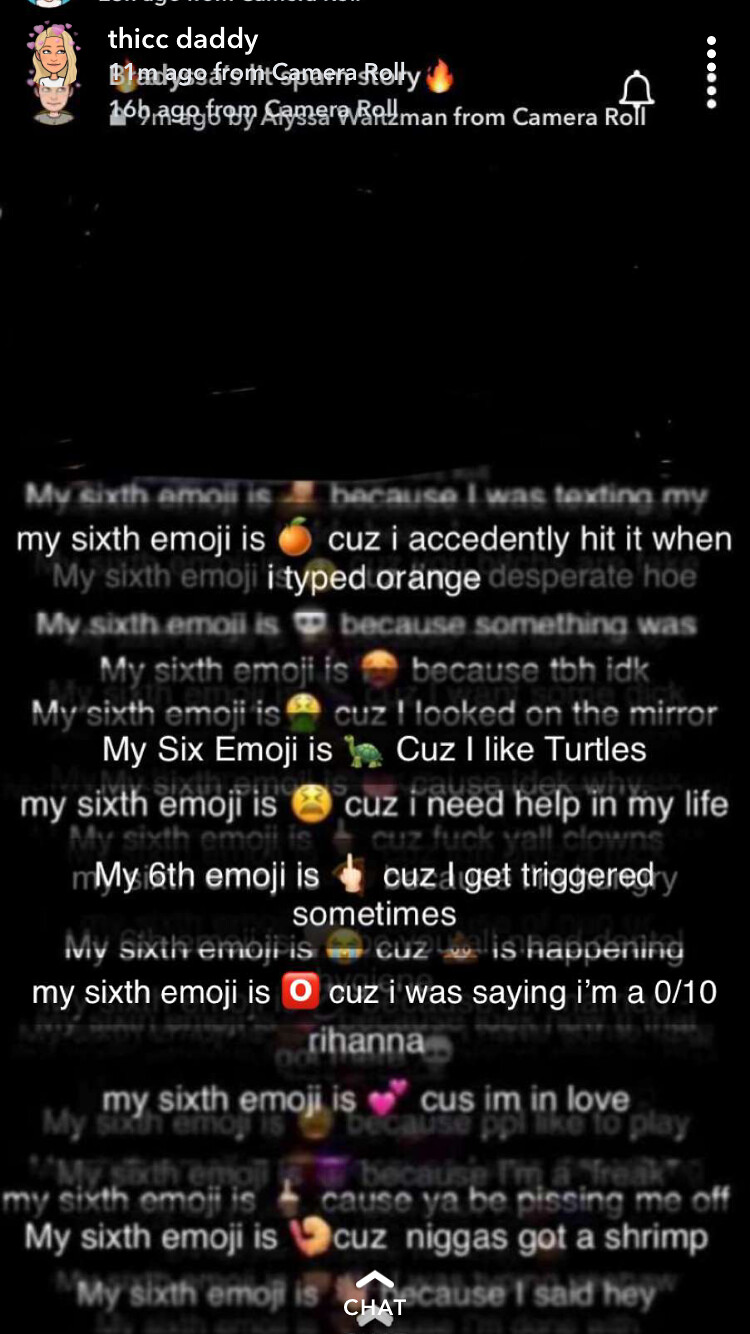The image depicts a screenshot taken on a phone, likely showing a series of posts or a chat sequence on a social media platform, possibly Twitter. The user, identified as "THICCDaddy," is engaged in a playful trend involving emojis. At the top of the screenshot, there is a cartoon image of a blonde female and a cartoonish boy, with "Camera Roll" and a fire emoji displayed. A bell icon and six vertical dots are also visible.

The central focus is a series of overlapping messages, each starting with "my sixth emoji is." The posts include various emojis followed by humorous or self-deprecating explanations: an orange (accidentally typed), a turtle (because "I like turtles"), a crying face (indicating a need for help), a middle finger (due to feeling triggered), a zero (self-assessment as "zero out of ten"), two hearts (expressing love), and a shrimp (using a racial slur in a jocular manner).

The text, in small white script, is largely clear against the black background despite some parts being blurred or overlapping. The repeated structure and varied explanations create a comedic montage reflecting the user’s interaction with emoji culture.